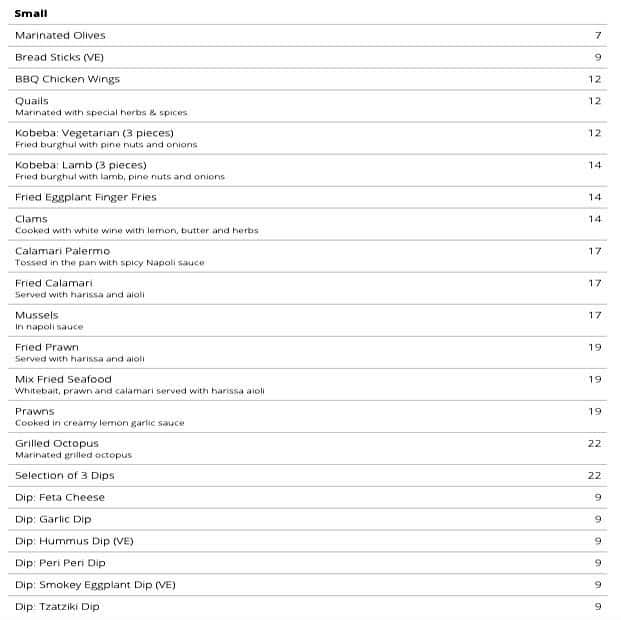In the image, we see a detailed menu list with various dishes and their descriptions. The items are as follows:

1. **Breadsticks (7)** - Simple yet classic, these breadsticks are featured at the top of the list.
2. **BBQ Chicken Wings (9)** - Succulent and savory, these wings are prepared with a rich BBQ sauce.
3. **Marinated Quails (12)** - These quails are infused with special herbs and spices for an extraordinary flavor experience.
4. **Kobeba, Vegetarian (12, 3 pieces)** - These vegetarian fried burgers are filled with pine nuts and onions.
5. **Kobeba, Lamb (12, 3 pieces)** - Similar to the vegetarian version but filled with lamb, pine nuts, and onions, offering a rich and savory taste.
6. **Fried Eggplants and Finger Fries (14)** - A delightful combination of crispy fried eggplants and golden finger fries.
7. **Clams Cooked with White Wine (14)** - These clams are delicately cooked in white wine with lemon, butter, and a hint of herbs for a flavorful finish.
8. **Calamansi Palamu (17)** - This dish features Calamansi tossed in a pan and cooked with a spicy Nepali sauce for a bold and zesty flavor.

Each dish is numbered and listed with corresponding prices to give a comprehensive description to the viewer.